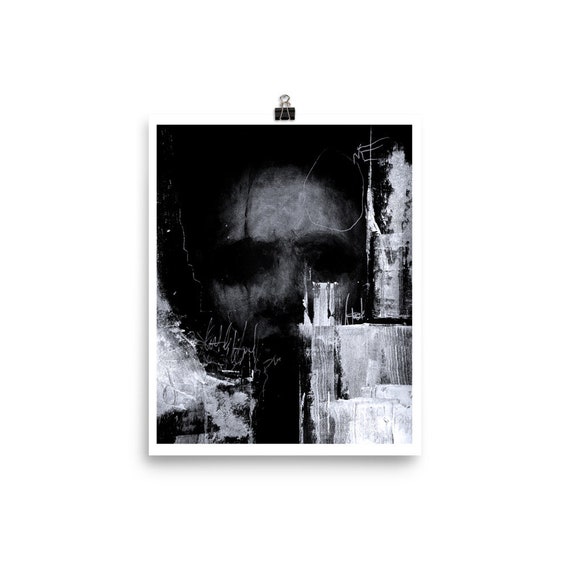In this eerie black-and-white image, a printed photograph is held up by a binder clip against a stark white background. The photograph itself is predominantly black, with enigmatic white smudges and streaks scattered throughout. In the bottom left and right sections, these smudges appear almost like melted wax or paint drips, lending a distressed, unsettling texture to the image. The top right corner features what looks like an abstract cylindrical object or an antenna-like shape made from smeared white markings.

At the center of this dark and haunting artwork, a ghostly face emerges from the shadows. The face is partially obscured, with visible features including a forehead bearing a scar, a nose, and lips, but the eyes remain dark voids, giving the visage a spectral and haunting feel. The face seems almost etched into the blackness, set against the white smudges that surround it. The overall effect is one of sinister mystery and abstract horror, as if the face is materializing from the abstract chaos of the white streaks and smudges.